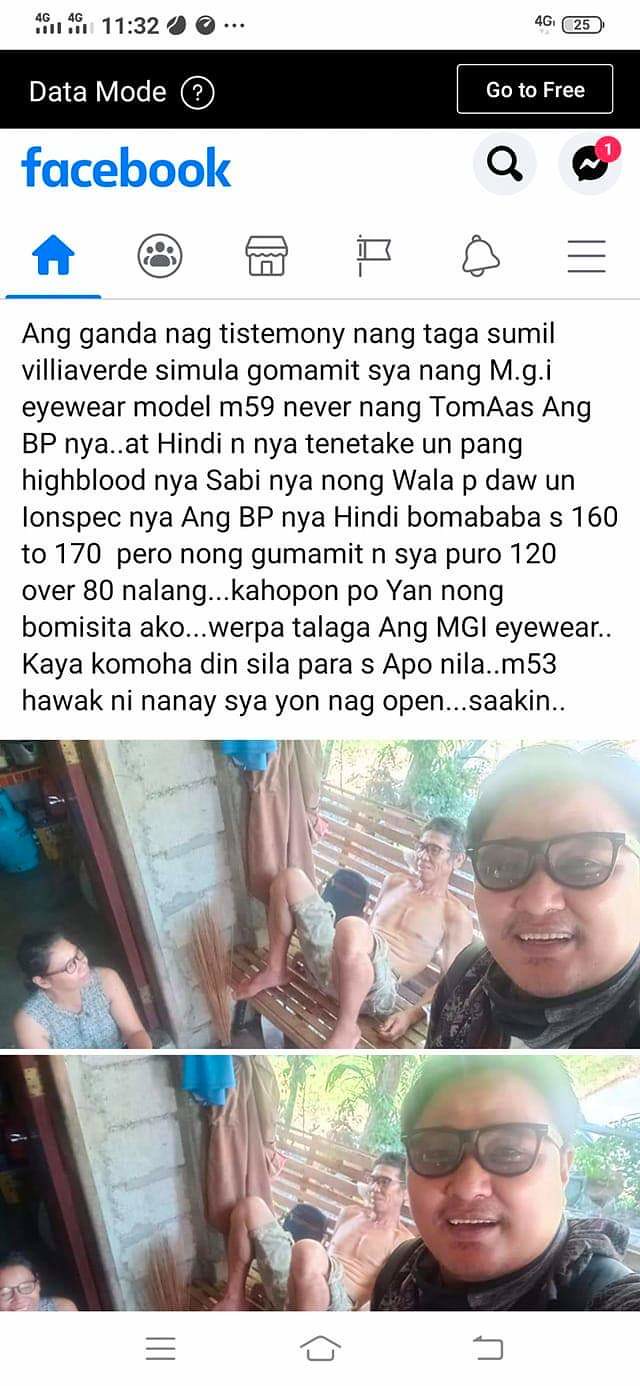This image is a screenshot from the Facebook mobile app. The top part of the screen displays typical smartphone icons: wireless or mobile data indicators, the time (11:32), and a battery meter. Below that, on a black banner, it reads "Data Mode ?" followed by "Go To Free." The familiar Facebook interface is below, featuring the Facebook logo, a search icon, and a messenger icon with a red notification bubble indicating "1" message. The navigation bar contains icons for Home, Friends, Marketplace, Groups, Notifications, and the menu.

The main content area shows a lengthy paragraph of text in a foreign language, mentioning words like "Anga, Ganda, Nanga," and "testimony." Below the text is a collage of two similar photos. The top image depicts a selfie with a man in the foreground and several people sitting on a wooden bench near a stone building with trees in the background. A woman with black hair, glasses, and a sleeveless blouse, appears to be talking to a shirtless, bespectacled man in khaki shorts. To the right, another man with sunglasses and a black top is visible. The second photo is almost identical, capturing a slight variation in their poses from just a moment later.